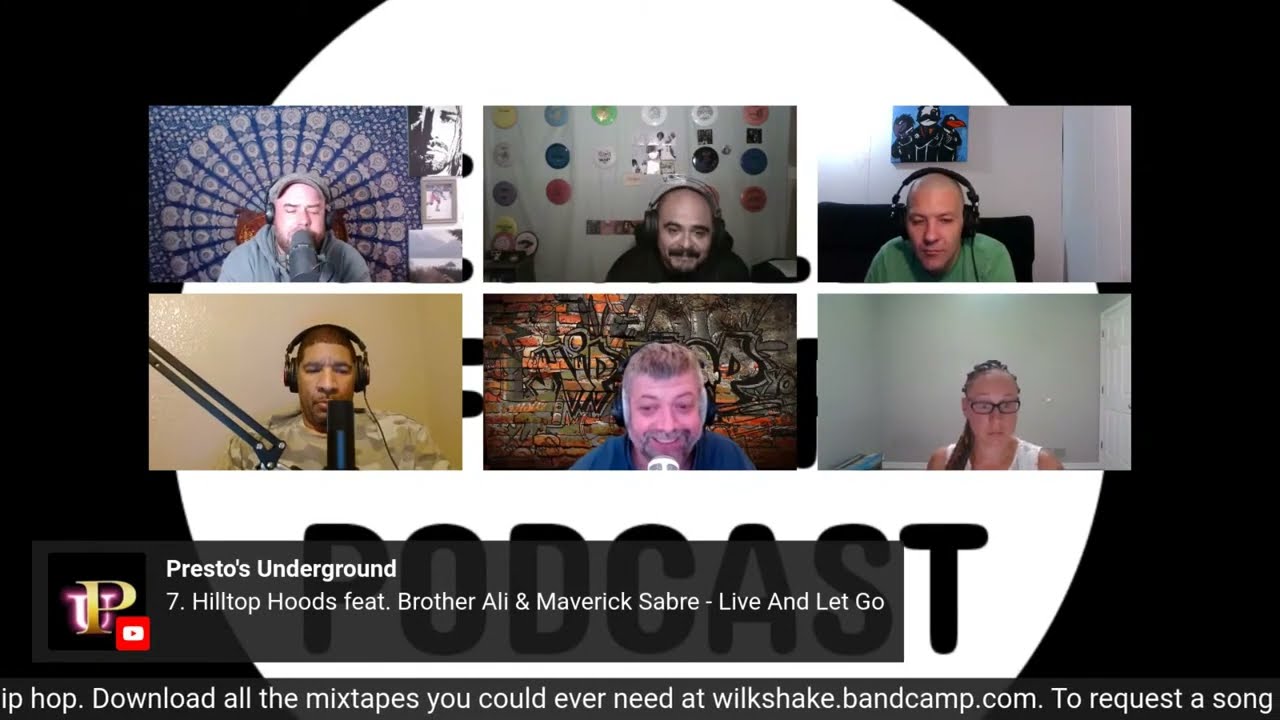The image is a colored screenshot from what appears to be a podcast hosted on YouTube, set against a solid black background with a prominent white circle at the center. Overlaid on the white circle are six equally-sized, horizontal rectangular panels, each depicting a participant of the podcast. 

The upper left panel features a stocky man wearing a hat, seated in front of a microphone with a gray background and an image of a circle behind his head. The central top panel shows a bald man in his late 20s or early 30s, sporting a mustache and wearing headphones, with a white wall and circular decorations behind him. The rightmost panel in this row reveals a man who appears to be slightly older, perhaps in his 30s, also wearing headphones and speaking into a microphone. He is seated in a dark red burgundy chair, with a white wall and a square photo hanging behind him, while dressed in a green T-shirt and leaning forward.

On the lower row, the leftmost panel shows a young black man with headphones and a microphone on a boom, against a tan eggshell background. He is wearing a light camouflage T-shirt. In the center panel of this row is a man in his early to mid-30s with gray hair and a gray beard and mustache. He leans forward towards a microphone, dressed in a blue T-shirt, with a multicolored, indistinct background behind him. The final lower right panel features a young woman in her 20s with light brown hair pulled back, wearing glasses and a white tank top, seated in front of a white wall.

Beneath these panels, the word "PODCAST" is written in black letters inside a gray bar. In the forefront, white sans-serif lettering spells out "Presto's Underground," followed by "7. Hilltop Hoods Fest. Brother Ali and Maverick Saber - Live and Let Go." To the left of this text is a logo resembling a capital 'P' next to the YouTube icon. At the very bottom of the image, more white text reads, "Download all the mixtapes you could ever need at wilkshake.bandcamp.com. To request a song."